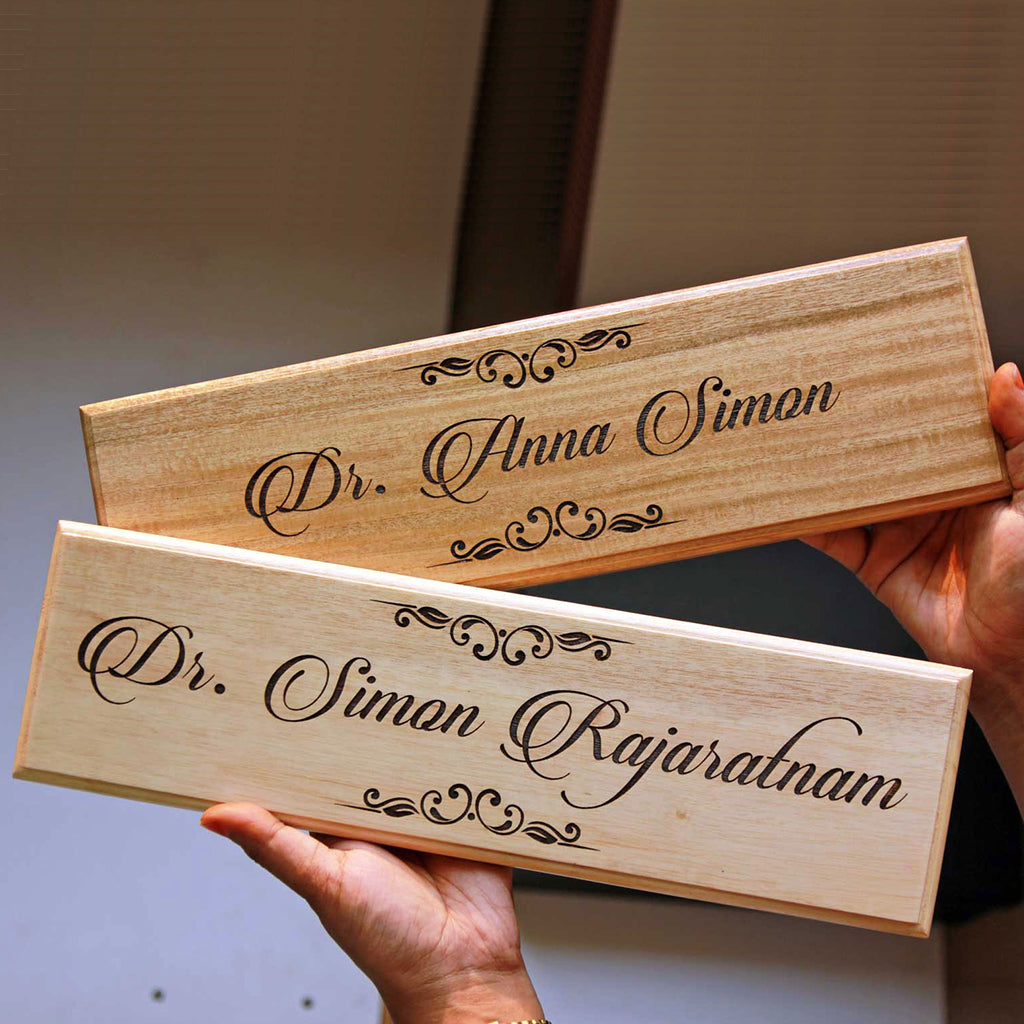This photograph features a pair of Caucasian hands holding two finely crafted wooden plaques against a slightly out-of-focus background, characterized by a white wall and a red banister at the top center. The primary focus is on the two plaques. In the left hand, a plaque with the text "Dr. Simon Rajarathnam" is displayed; it is adorned with intricate floral etchings above and below the name, which is written in a fancy cursive script in black. This plaque, made from lighter wood, stands out for its detailed craftsmanship. In the right hand, another plaque of a slightly darker wood showcases "Dr. Anna Simon," also inscribed in black cursive with similar elegant floral designs framing the top and bottom. Both plaques are identical in size and horizontal shape, likely intended for professional use, possibly to be displayed in a doctor's office or on a desk. The meticulous detail and harmonious design elements suggest a partnership or association between the two individuals.